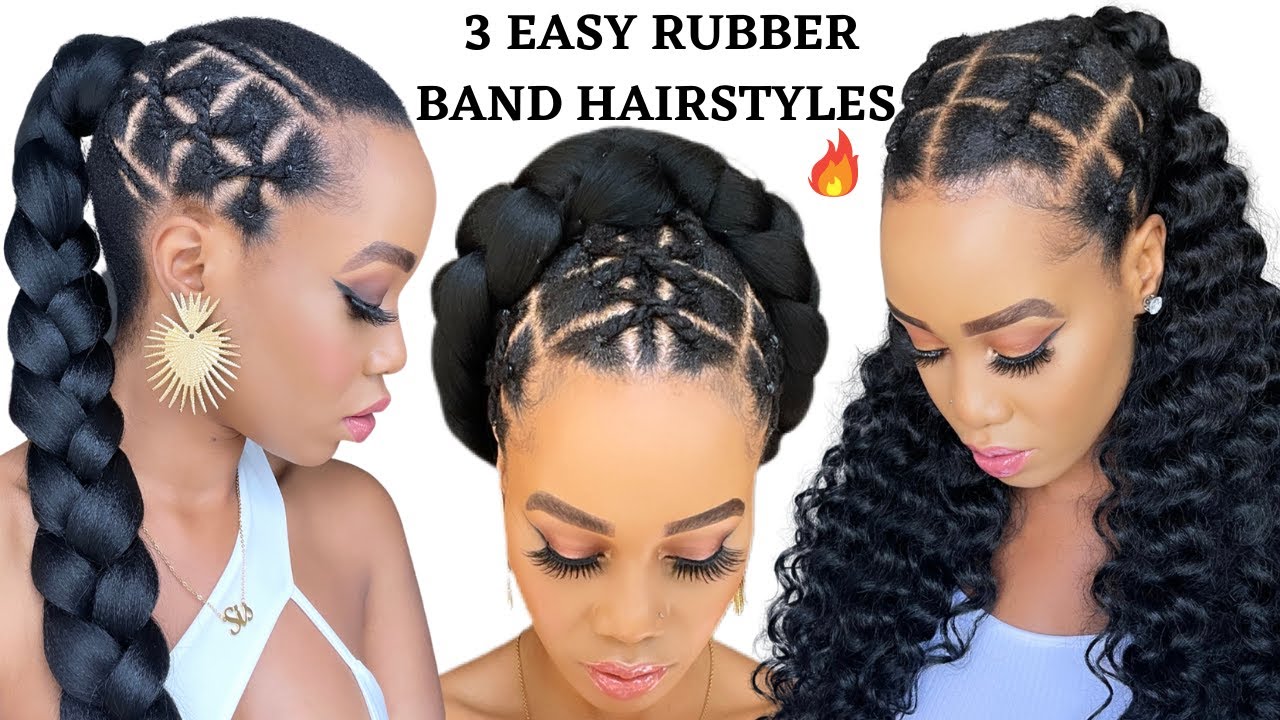The image is an advertisement showcasing three easy rubber band hairstyles for women with intricate braids. At the top, in black text against a white background, it reads "Three Easy Rubber Band Hairstyles". Directly beneath this text, to the right, is a flame emoji. The image features three women, possibly the same model in different poses, all with long eyelashes, pink lipstick, and drawn-on eyebrows. They have an olive complexion and are looking down, highlighting their detailed hairstyles.

The woman on the left, in a side profile, is adorned with purple eyeshadow, a long braid with X patterns, a gold heart-shaped earring with spikes, a revealing white one-shoulder dress, and a necklace that appears to say "SIS". The center model, visible from the head and shoulders, wears pink eyeshadow and flaunts a complex braid pattern on top of her head with a braid looped around the back. The right model, dressed in a blue shirt with pink eyeshadow, has wavy hair fashioned in a grid-like pattern at the top, and her earring seems to have a crystal design. All elements are presented on a clean, white background, emphasizing the hairstyles and makeup of the women.